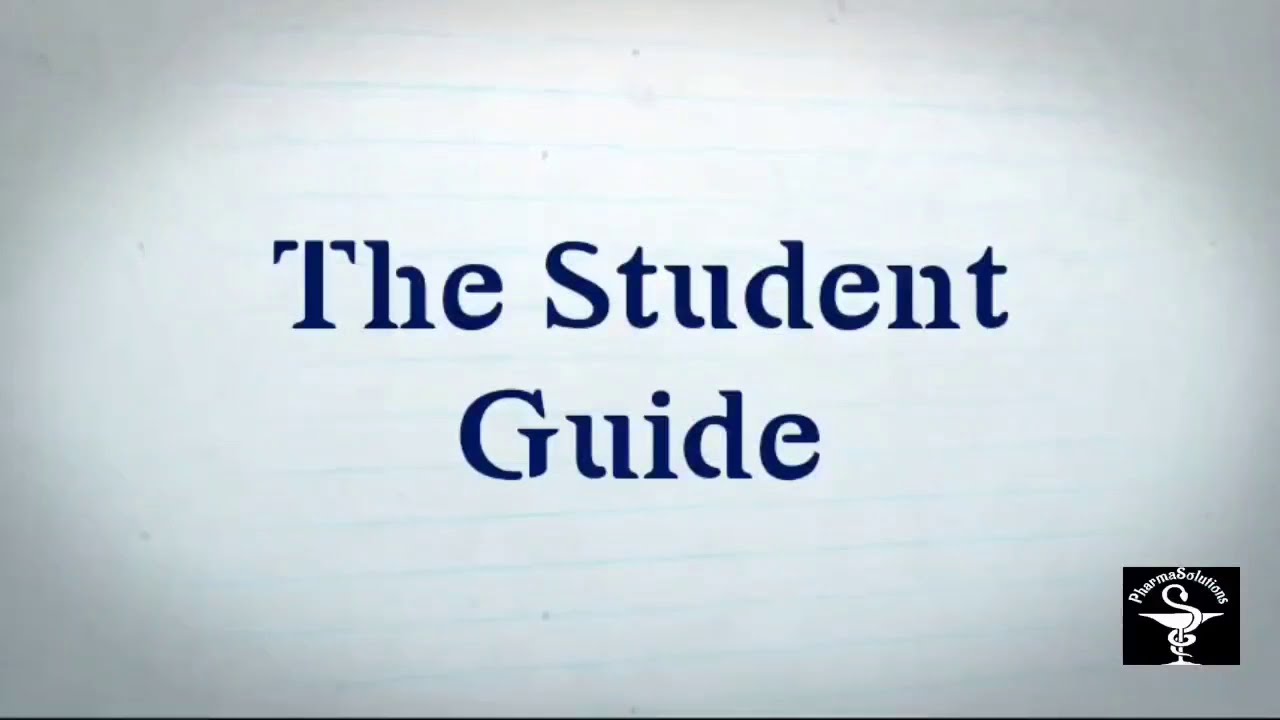The image features a cover or first page of a student guide with a muted grayish background resembling a student's notebook paper, adorned with faint, thin horizontal blue lines that become more vivid towards the center. The corners of the background appear darker, gradually lightening towards the middle. Centered in dark blue typewriter-style font are the words "The Student" on the top line and "Guide" on the second. Notably, several letters, excluding 'E' and 'T' and ‘S’, have subtle cuts giving a spatial effect between them.

In the bottom right corner, there is a detailed white symbol outlined in black, resembling a pharmacy insignia. This emblem features a serpent coiled around a shape similar to a genie lamp with an extended handle. The serpent wraps around the lamp one and a half times and then forms an S-shape with its body, its head curving downwards. Above this symbol, the words "Pharma Solutions" are written in a white arch, contrasting against the overall darker background.